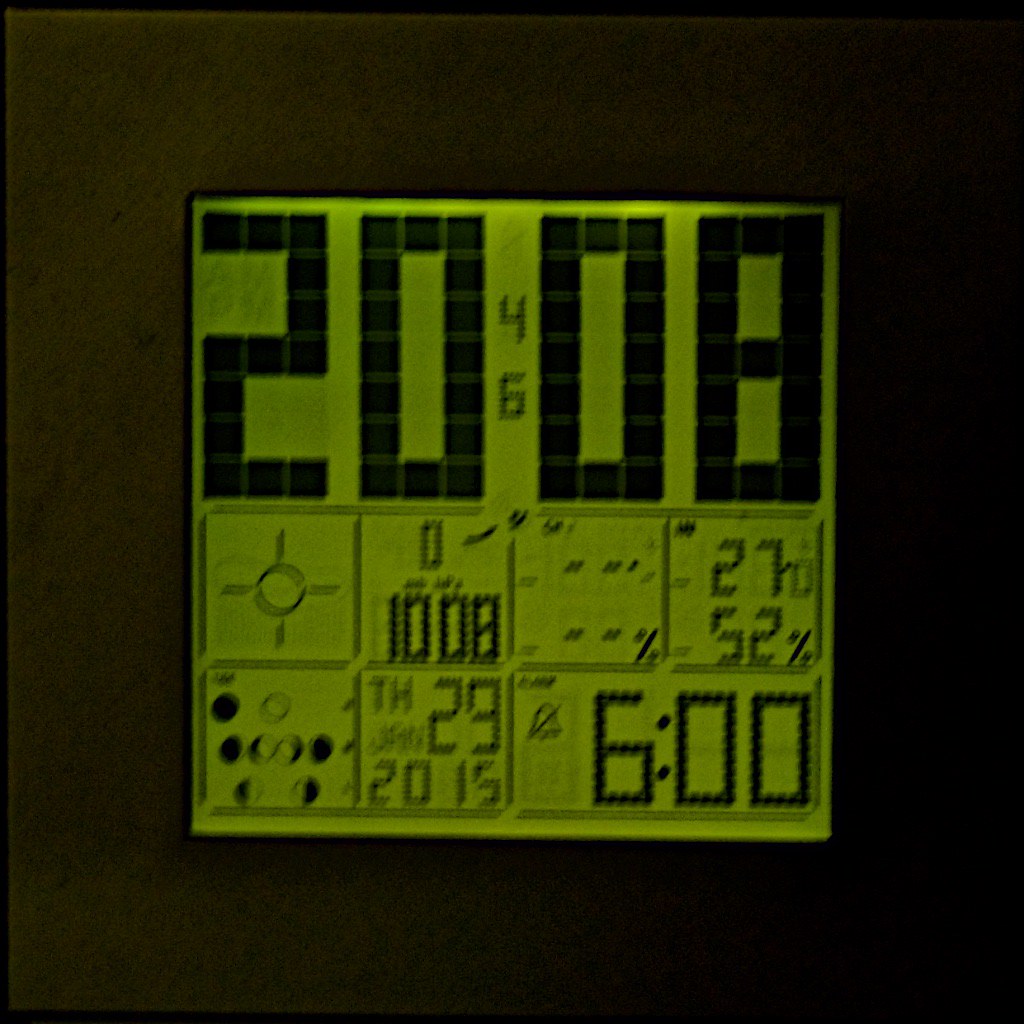Displayed against a black background, the image showcases a square frame centrally positioned. Within this frame lies a smaller, digitally illuminated square with a green backlight and black display. Dominating the top half of the digital display are large numbers reading "2008." Nestled vertically between the two zeros are smaller numbers, "4" above and "6" below. The bottom half of the display is segmented into eight distinct boxes, arranged in two rows of four. Each of these boxes contains various numbers and symbols, adding to the intricate detail of the digital readout.